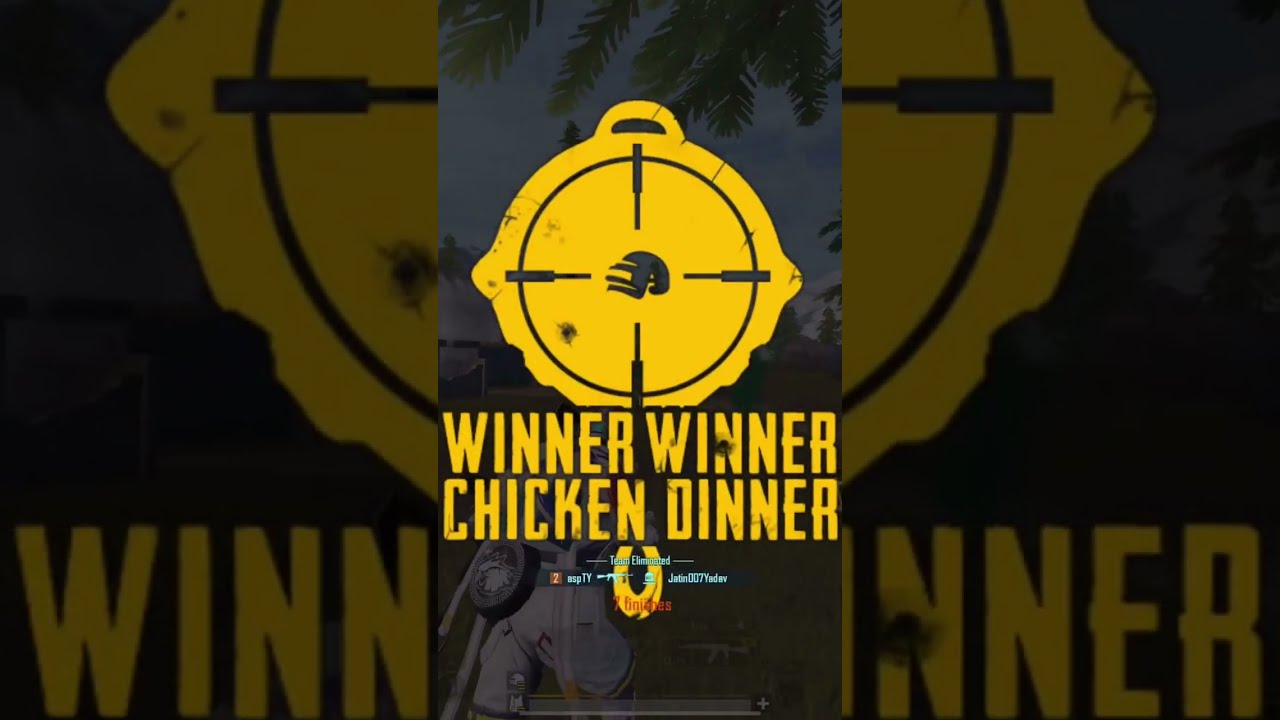The image is a vertically oriented, cell phone-style graphic depicting a promotional or informational announcement related to a video game. Central to the design is a large, round emblem resembling a lock with a handle at the top and a border that appears bumpy at the bottom. Inside the emblem is a black circle outline with four inward-pointing indicators at the 12, 3, 6, and 9 o'clock positions, resembling crosshairs targeting a slightly indiscernible object or shape that looks like a helmet. Right below the emblem, in prominent yellow all-caps font, is the text "WINNER WINNER CHICKEN DINNER." Below this text, there are additional lines of blue and red font that are too small to be legible. The image's background features a faded and zoomed-in version of the central graphic, creating an immersive visual effect.